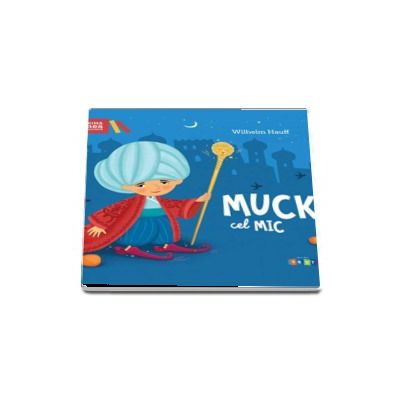The image features a children's book titled "Muc-Kal-Mik" by William Moot, with bright, white, bold lettering. The book cover predominantly displays a child in full Arabian attire: a red robe, white turban, blue pants, and long, pointed purplish shoes, holding a bright gold staff. The backdrop is a vivid blue, adorned with Arabian-style houses and towers, and a large white moon centered on the page. The child and the title occupy most of the cover, which lies flat against a stark white background, positioned perfectly in the center of the image. The colors on the cover include shades of blue, red, yellow, light blue, and orange, suggesting it is a visually striking children's book.